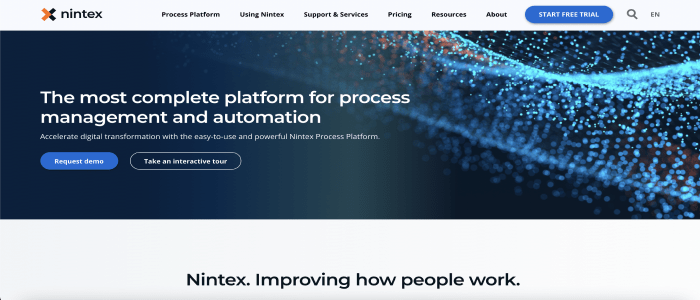The screenshot displays the homepage of a website. At the very top, there is a light gray border. On the left-hand side, a logo is visible, which resembles an 'X' with the left half in peach color and the right half in black, split down the middle. Next to the logo, there is text in lowercase letters that reads "nintex."

To the right of the logo and text, a navigation menu is displayed in black letters with the following items: "Process Platform," "Using Nintex," "Support and Services," "Pricing," "Resources," and "About." Adjacent to the "About" link, there is a blue button with white text that reads "START FREE TRIAL" in all capital letters. To the right of the button, there is a magnifying glass icon, presumably for search functionality, followed by the text "EN" in dark gray letters.

Beneath this top section, the header image spans the width of the page and features a technical blue design. The left side of the image is solid blue, while the right side showcases glowing dots and lines, giving it a high-tech appearance. Positioned on the left side of this image, the heading text in white reads, "The Most Complete Platform for Process Management and Automation." Below this, in smaller white letters, is the subheading: "Accelerate digital transformation with the easy-to-use and powerful Nintex process platform."

Underneath the heading and subheading, to the left, there is a blue button labeled "REQUEST DEMO," and to the right, another button with a white outline and dark blue background that says "TAKE AN INTERACTIVE TOUR" in white text.

Further down the page, there is a block section with a light grayish-white background. This block contains space at the top and, in the middle, the black text reads, "Nintex: Improving How People Work." Below this statement, the section transitions into white space which likely signifies the end of the visible portion of the screenshot.